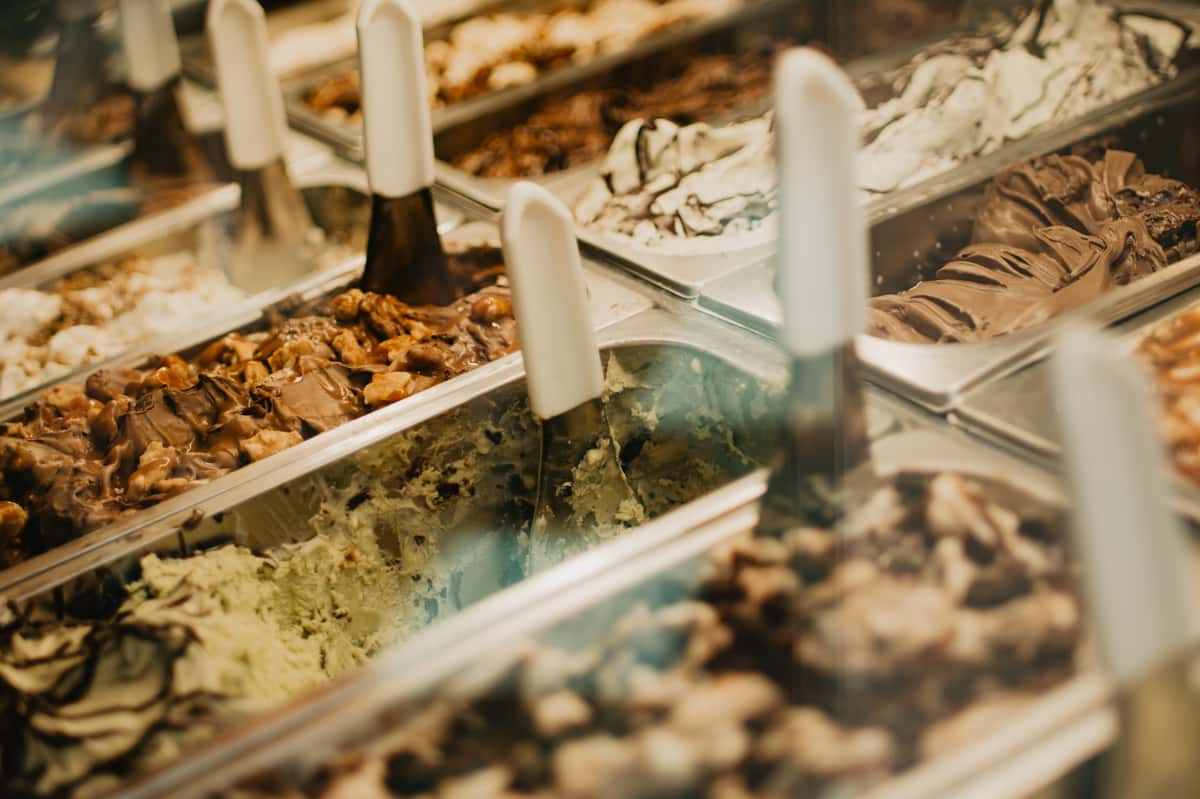The close-up image showcases an assortment of stainless steel rectangular serving trays, each filled with various flavors of ice cream or gelato. Each tray is equipped with a serving spoon that has a distinctive white handle. The trays feature a vibrant array of colors and textures: a green-hued ice cream, possibly pistachio, which is half-empty; several trays with chocolate ice creams, some containing nut pieces; and a white ice cream with prominent brown stripes that resemble fudge ribbons. Additionally, a tray with a chocolate and vanilla swirl can be seen in the top right corner, alongside a few other full containers of different flavors.